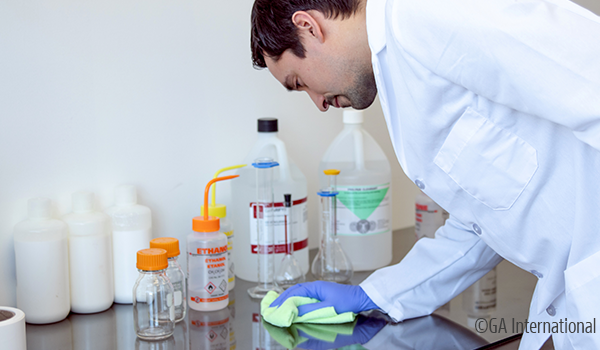This photograph captures a man in a white lab coat with buttons down the middle, meticulously wiping down a reflective laboratory bench with a neon green towel held in his blue latex-gloved right hand. The man, who has short brown hair and a slight beard, appears focused as he cleans up what might be a chemical spill. The lab bench, which has a pewter metal finish, is cluttered with various laboratory items including several beakers and measuring containers. Prominent among them are jugs of clear liquids, possibly alcohol or ethanol, and bottles with orange caps, clearly labeled as ethanol. Also visible are other containers, some holding unknown powders with different colored lids, including yellow and orange screw tops, and two larger bottles in the background, one with a black lid and the other with a white lid. The scene is set against a backdrop featuring additional lab equipment, emphasizing the scientific environment. The image conveys a sense of meticulous care and organization typical in laboratory settings, underscored by the subtle watermark "copyright GA International" in the bottom right corner.